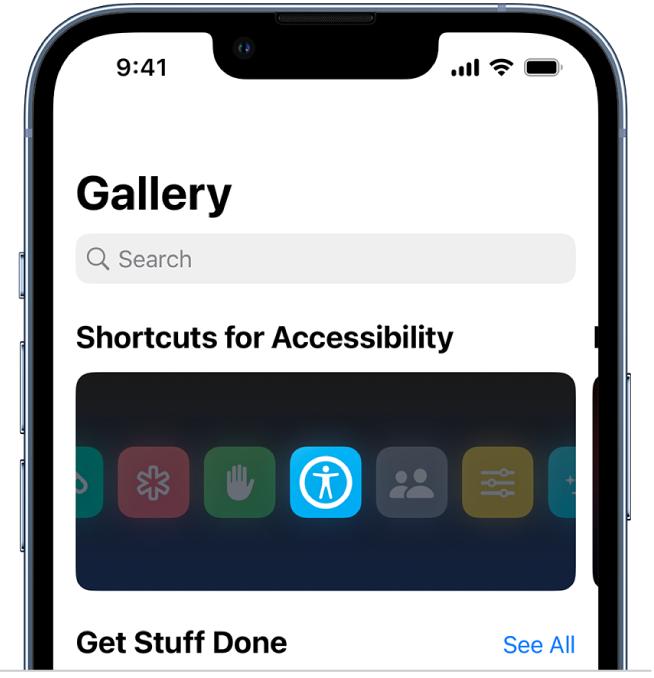This image appears to be a mock-up of an iPhone screen displaying the interface of a gallery app. At the top of the screen, the word "Gallery" is clearly visible, followed by a search bar just below it. Beneath the search bar, there are several shortcut icons dedicated to various functions, with a central icon representing accessibility—depicted as a generic human figure in a Vitruvian Man pose within a circle. Further down the screen, there's a section labeled "Get Stuff Done," accompanied by a link that says "See All." The specifics of the app's functionality remain unclear, but it seems to integrate multiple features for viewing, editing, or organizing content, as suggested by the assorted icons and sections.

The phone mock-up includes the typical design elements of an iPhone, such as an outline with a notch at the top of the screen. The status indicators at the top show a time of 9:41, a fully charged battery, strong cellular signal, and robust Wi-Fi connectivity.